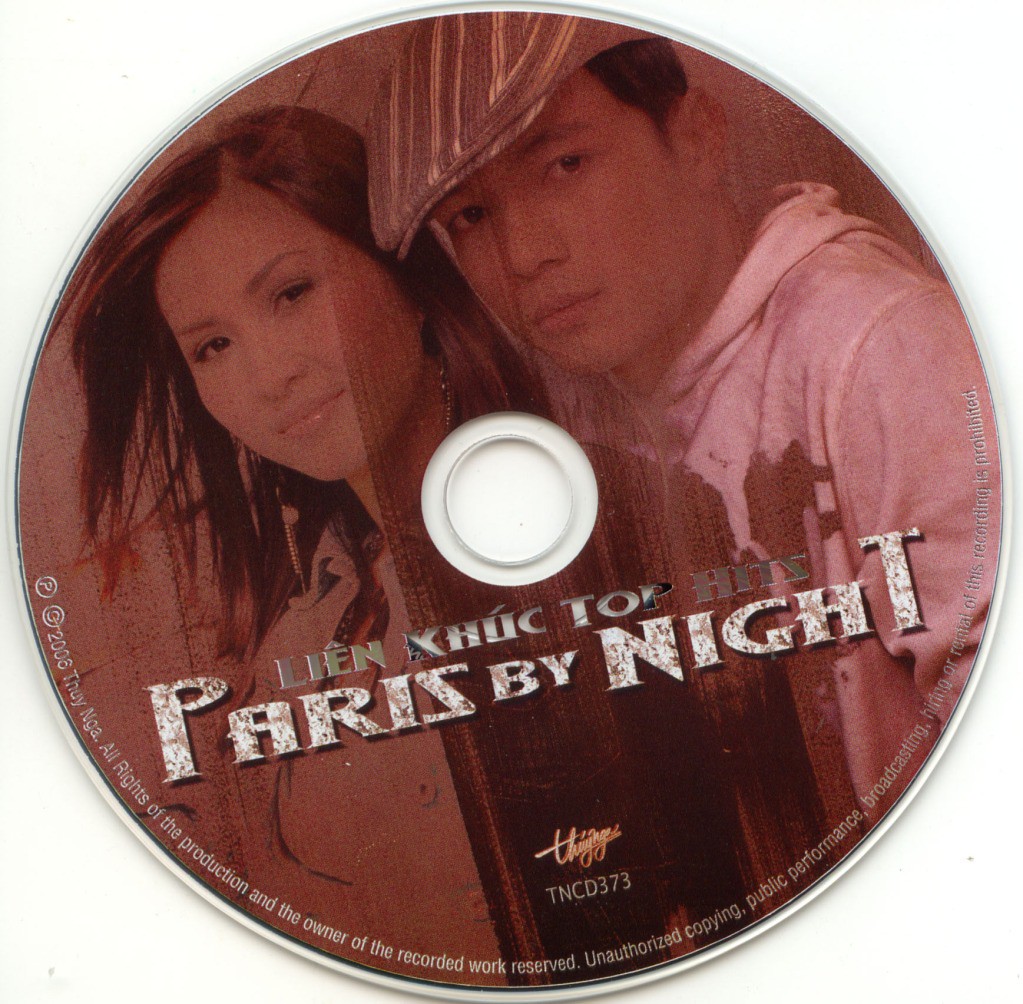This photograph showcases a music CD titled "Paris by Night," prominently displayed in bold white text across the top of the disc. Above the title, it reads "Lien Khuc Top Hits," indicating the album category. The CD features a teal and reddish hue background, adding a textured appearance. Centrally, there's a vibrant image of a Caucasian man and woman, both dressed in white and smiling at the camera. The woman, with her long, dark brown hair, appears to the left, while the man, clean-shaven and wearing a white hoodie and a golf cap, stands to her right. Additional text on the CD includes "TN-CD-373" and a copyright declaration: "©2008, Theo Nigga. All rights of the production and the owner of the recorded work reserved. Unauthorized copying, public performance, broadcasting, hiring, or rental of this recording is prohibited."